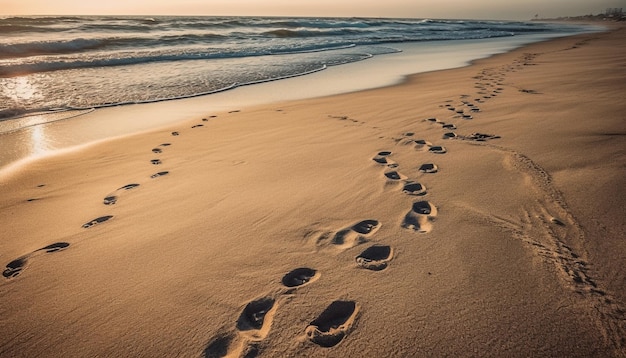In this evocative beach scene, the golden tan sand stretches along a serene coastline, appearing soft and fine-grained, unmarred by pebbles. Multiple footprints traverse this sandy expanse, creating a narrative of movement—one prominent set meanders parallel to the foamy waves lapping at the shore, while another, smaller set curves toward the water before veering back. The tranquil ocean, its waves crowned with grayish-white foam, extends into the distance, gently approaching the shore. The sunlight, possibly from a setting or rising sun, casts a mesmerizing orange glow atop the water, enhancing the scene with a warm, ethereal light. Accompanying this are the reflections of light that subtly dance on the water's surface, suggesting the day's end. The far stretch of the beach remains unspoiled, only faintly dotted with distant buildings, underscoring the vast tranquility of this pristine seascape. A slight hint of pink in the darkening sky adds to the tranquil beauty, blending harmoniously with the bluish-gray hues of the ocean, ultimately capturing a scene of serene, natural elegance.